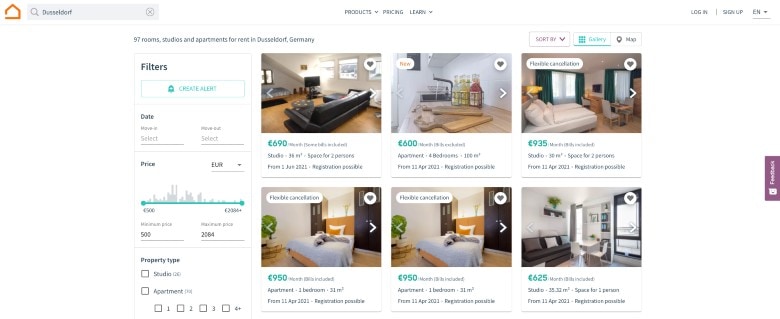This image appears to be a screenshot of a rental property search website. In the upper left corner, there's a brown outlined icon resembling a house, indicating the site's logo. Immediately to the right of the logo is a search bar. Centered at the top are dropdown menus labeled "Products," "Pricing," and "Learn." On the far right, there are options for "Login," "Sign Up," and a dropdown menu labeled "Ian."

The main portion of the image features a grid layout displaying two rows of property thumbnails, with three images in each row, showcasing apartments available for rent. On the left side of the page, there is a vertical sidebar that starts with filter options. Below the filters is a button labeled "Create Alert." Further down, there are fields to enter a date range, a price range, and a property type selection, offering options of "Studio" or "Apartment."

In the images of the apartments on the right side of the page, three of the listings display banners indicating they have flexible cancellation policies. Additionally, each property image has a heart icon in the top right corner, allowing users to favorite the listings.